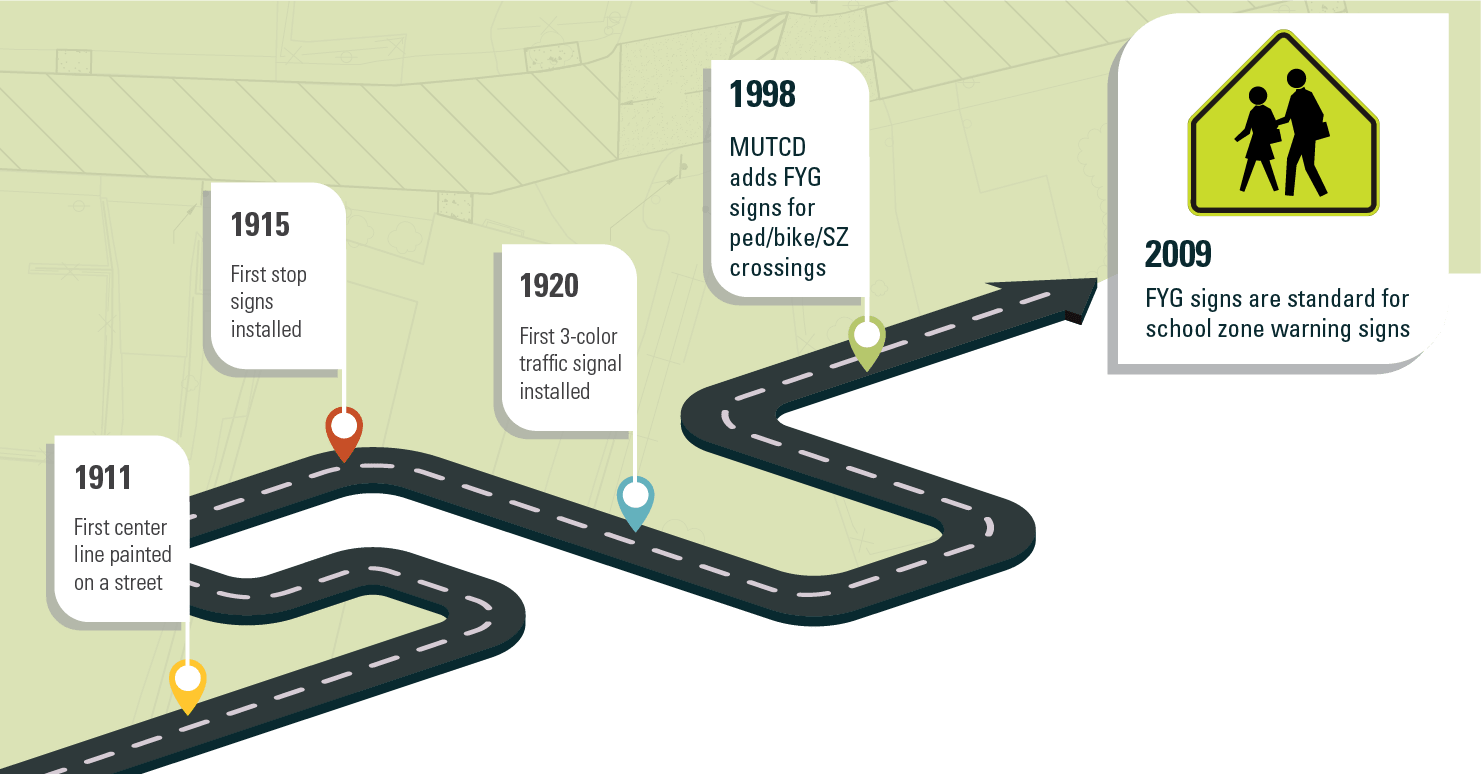The illustration is an informational poster depicting the evolution of road safety measures over time. A black roadway, marked with a white dashed center line, winds from the bottom left to the top right of the image. The road is bordered by a greenish tint suggestive of lot lines, with several colored waypoints marking historical milestones. Starting at the bottom left, a yellow waypoint is accompanied by a text box stating, "1911: First center line painted on a street." Further along, a red waypoint notes, "1915: First stop sign installed." Continuing down the road, a blue waypoint reads, "1920: First three-color traffic signal installed." Near the end of the road, a yellow-green waypoint highlights, "1998: MUTCD adds FYG signs for pedestrian, bike, and school zone crossings." The final waypoint showcases a familiar yellow school crossing sign with black figures of an adult and a child with a backpack, noting, "2009: FYG signs are standard for school zone warning signs."